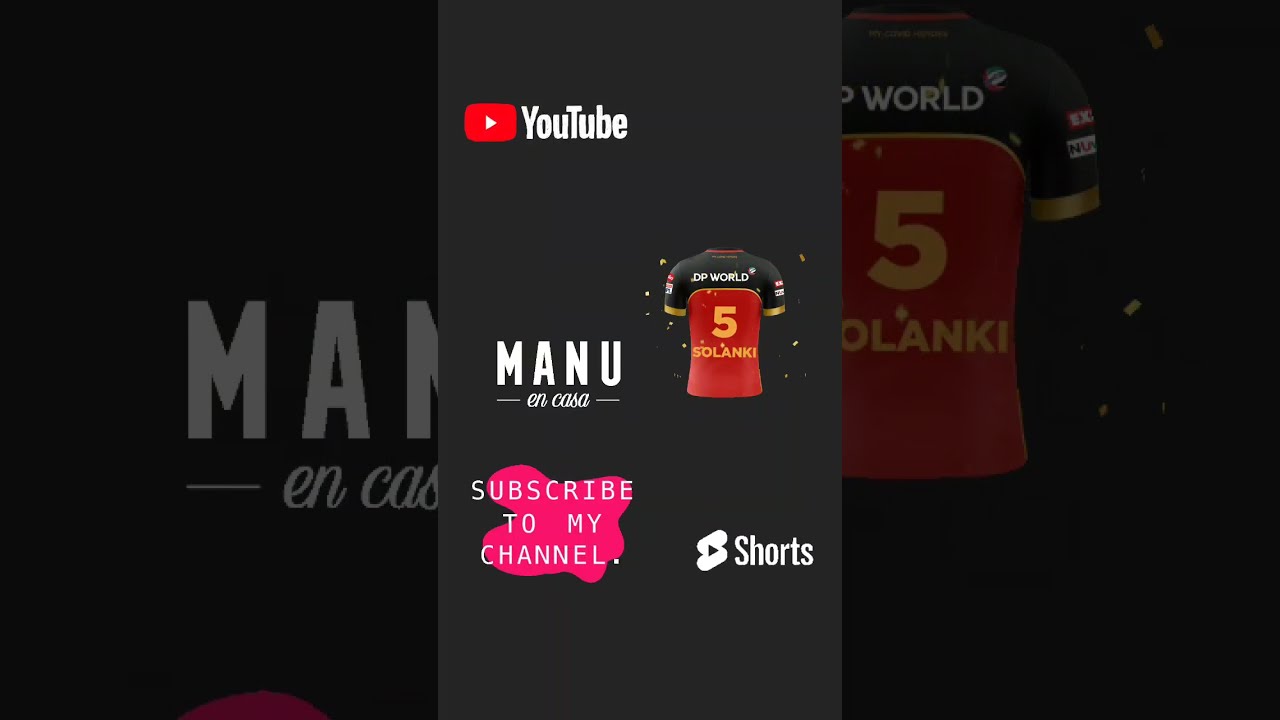The image appears to be a promotional screenshot from a YouTube stream. It features a dark gray, vertical portrait-mode banner divided into three panels. The most prominent central panel displays the YouTube logo at the top left, which includes the iconic red square with a white play button followed by the YouTube text. Right below it, large white text reads "Manu," with "En Casa" written in italics beneath it, separated by lines, suggesting a creator's name.

To the right of this text is a sports jersey, predominantly in red with black shoulders. The jersey bears the yellow number 5 with the name "Solanke" written at the bottom and "DP World" emblazoned in white across the top. Below "Manu En Casa," a pink, blobby background contains the white text, "subscribe to my channel." At the bottom right, the YouTube Shorts icon, an 'S' shape formed by two angled ovals with a play button in the center, is displayed.

The left and right sides of the image are filled with zoomed-in portions of the central elements, likely done to extend the portrait image into a landscape-friendly format.